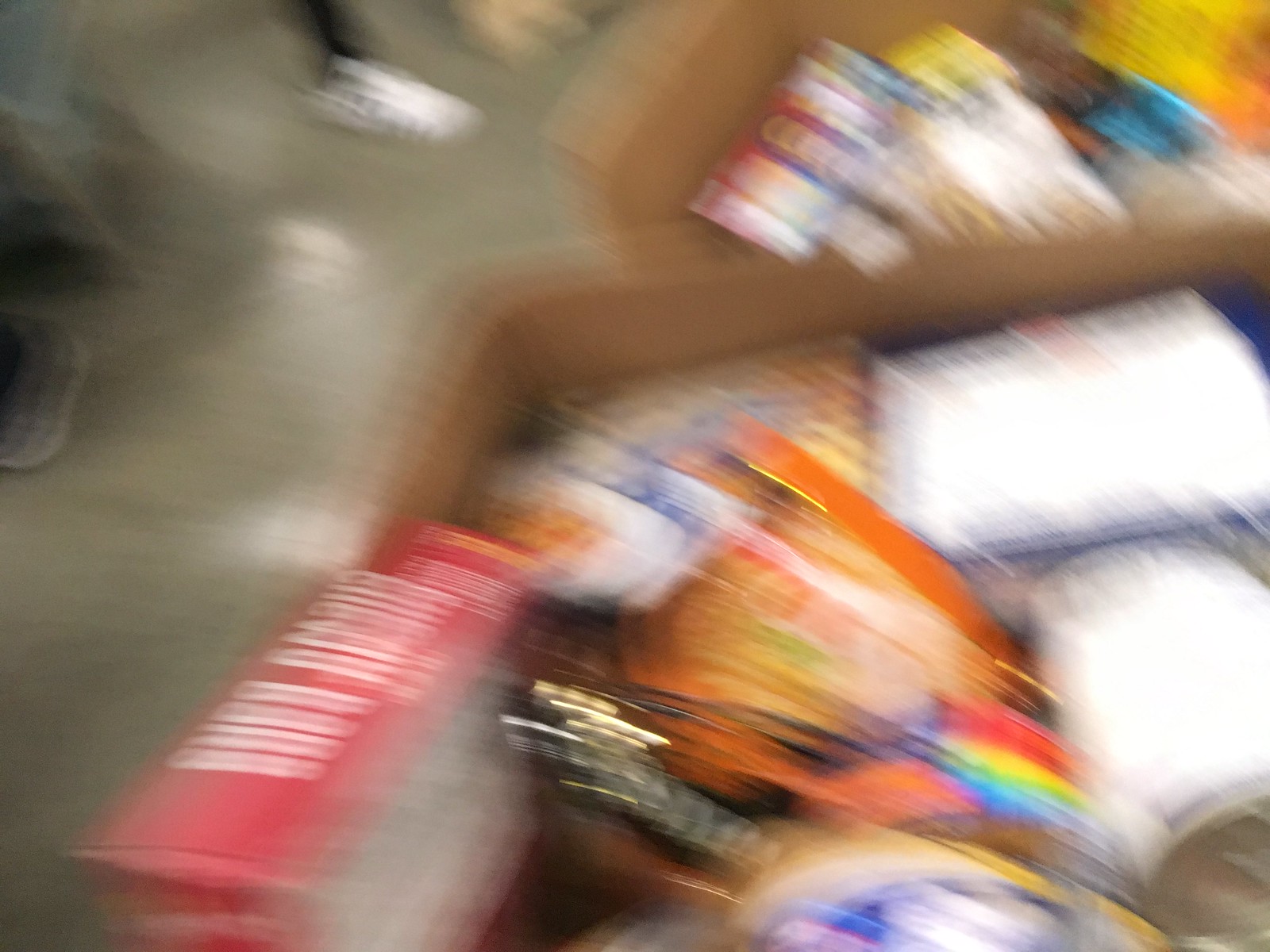A photograph depicts a collection of groceries inside either brown paper bags or cardboard boxes. The image is highly blurry, suggesting that the photographer may have been in motion or accidentally dropped their camera or phone. Despite the blur, brightly colored groceries stand out, including what seem to be vitamins and various boxed snacks. In the upper right corner, the foot of an individual wearing white sneakers is partially visible. The floor of the setting appears to be made of dark gray concrete, which is shiny and reflective, capturing the light from above.